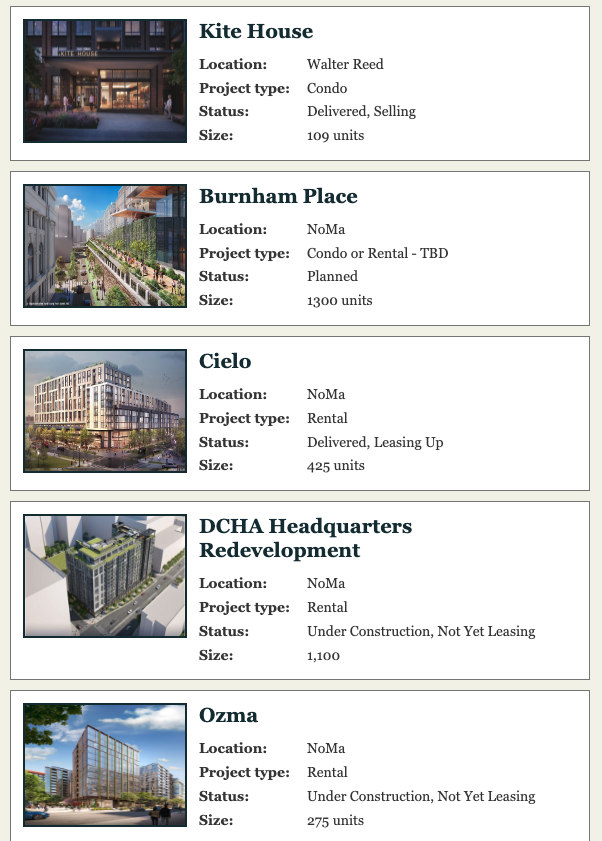### Detailed Caption for Vertically Aligned Locations Image

The image features five different locations, arranged vertically against an off-white background. The locations themselves are detailed on an off-white backdrop as well. The titles are displayed in a dark teal-blue color. Below is a detailed description of each location:

1. **Kite House**
   - **Location**: Water Road
   - **Project Type**: Condo
   - **Status**: Delivered
   - **Size**: 109 units
   - **Description**: The image shows a large condo building with a prominent, large window at the bottom, through which a bit of the interior can be seen. There is a spacious entryway visible as well.

2. **Burnham Palace**
   - **Location**: Noma
   - **Project Type**: Condo or Rental (TBD)
   - **Status**: Planned
   - **Size**: 1300 units
   - **Description**: This depicts a towering apartment building reaching into the sky, situated in a very busy area. The sky and other surrounding buildings are visible.

3. **Cielo**
   - **Location**: Noma
   - **Project Type**: Rental
   - **Status**: Delivered, Leasing Up
   - **Size**: 425 units
   - **Description**: The image shows a large silver apartment building with a view of the sky and streets around it.

4. **DCHA Headquarters Redevelopment**
   - **Location**: Noma
   - **Project Type**: Rental
   - **Status**: Under Construction, Not Yet Leasing
   - **Size**: 1100 units
   - **Description**: The depicted building is a gray structure amidst construction, with surrounding buildings shown as white, resembling a 3D program illustration.

5. **Ozma**
   - **Location**: Noma
   - **Project Type**: Rental
   - **Status**: Under Construction, Not Yet Leasing
   - **Size**: 275 units
   - **Description**: The image shows a large building with shiny glass windows. The surroundings include similar buildings, a cloudy blue sky, some trees, and a street.

Each image on the left complements the description with a visual representation of the respective buildings and their environments.